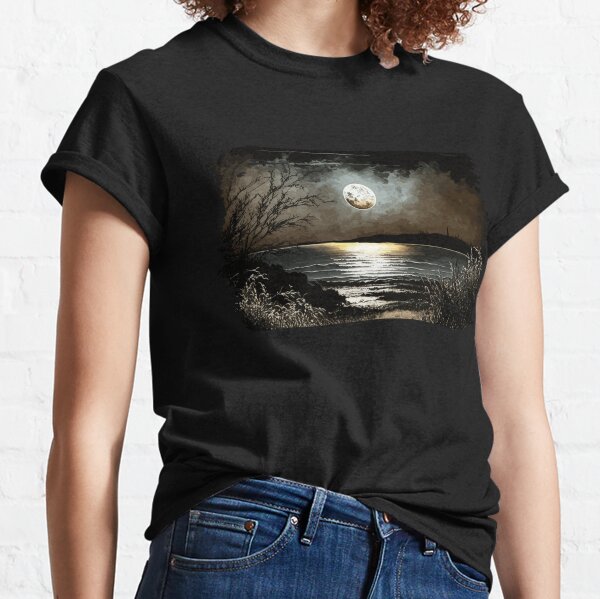In the photograph, a young woman is modeling a black, short-sleeved baby doll t-shirt, partially tucked into dark navy blue jeans. She is Caucasian with fair skin and brown curly hair, although her face is not visible as the image focuses solely on her torso. The black t-shirt prominently features a rectangular graphic of a moon rising over a body of water at night, with trees, reeds, and other plants depicted on the riverbank. The shirt is tucked in at the front while the sides hang loose. The background is stark and featureless, contributing to an overall clean and minimalistic presentation likely intended for an online store or advertisement.